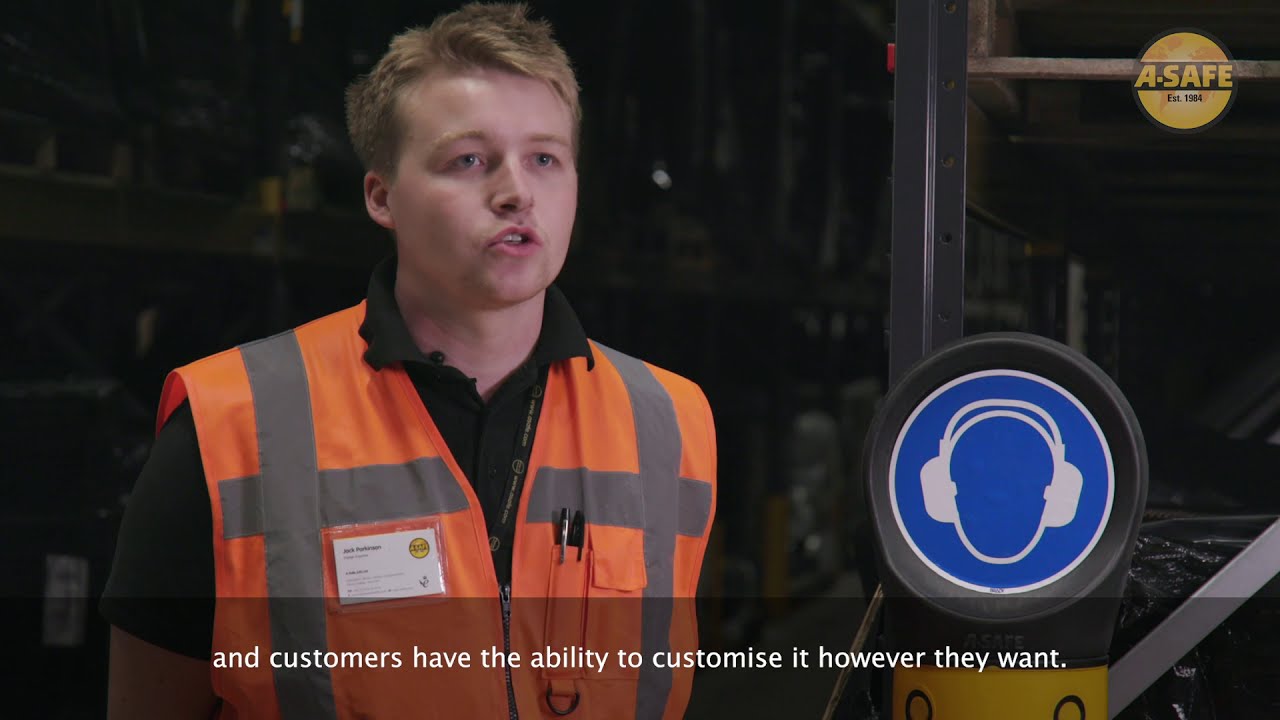In the image, a Caucasian man stands towards the left, sporting short sandy blonde hair, an orange and gray safety vest, and a black collared shirt. His vest features a name tag identifying him as Jack Parkinson and a pen pocket with two pens. The man appears to be talking, his lips pursed in speech. To the right of him is a blue circular safety icon depicting a head wearing ear protection. Further to the right, the backdrop reveals warehouse storage rows and dividers. The top right corner of the image displays a circular logo in yellow and black that reads "A-SAFE, established 1984." At the bottom, a white text states, "customers have the ability to customize it however they want." The setting suggests an advertisement, likely promoting safety equipment or services.